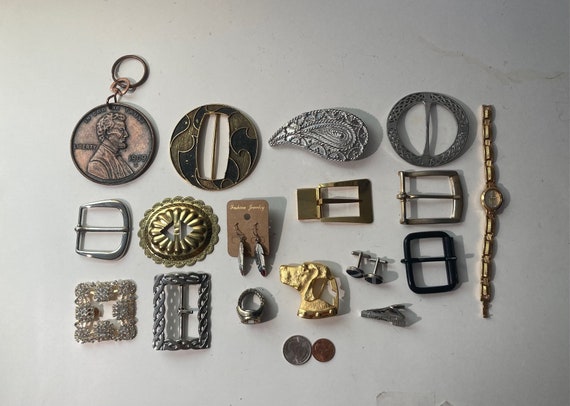This is a meticulously arranged photograph of various trinkets and small items displayed on a light gray background. In the top-left corner, there's an American penny dated 1909 with an attached keychain loop, making it resemble a pendant. To the right of the penny, there's a black circular object with a gold design and a central rectangular opening, followed by a teardrop-shaped silver item. Further right, a round silver object with a central hole and a vertical silver rectangle continues the arrangement.

Below these items on the second row, starting from the left, there's a silver belt buckle. A golden flower-shaped object is placed next, followed by a brown rectangular piece with two silver oval earrings hanging from it. Subsequent items include a gold belt buckle with a rectangular side and a brass-tinged belt buckle. Dominating the right side of the frame is a small watch featuring gold segmented bands and a matching gold face.

In the bottom row, the arrangement begins with an intricate shiny square design, followed by an ornate matte silver Celtic knot-style belt buckle. Next, there's an upside-down silver ring, a gold icon of a dog facing left, and two dark-faced cufflinks. Completing this row is a black belt buckle.

At the very bottom right of the image, there are two coins: an American quarter and an American penny, which are notably smaller compared to the other objects. Additionally, there's a small silver object that appears to be rectangular or triangular in shape. The assortment conveys a diverse collection of jewelry pieces and belt buckles, showcasing variations in gold, silver, and bronze hues.